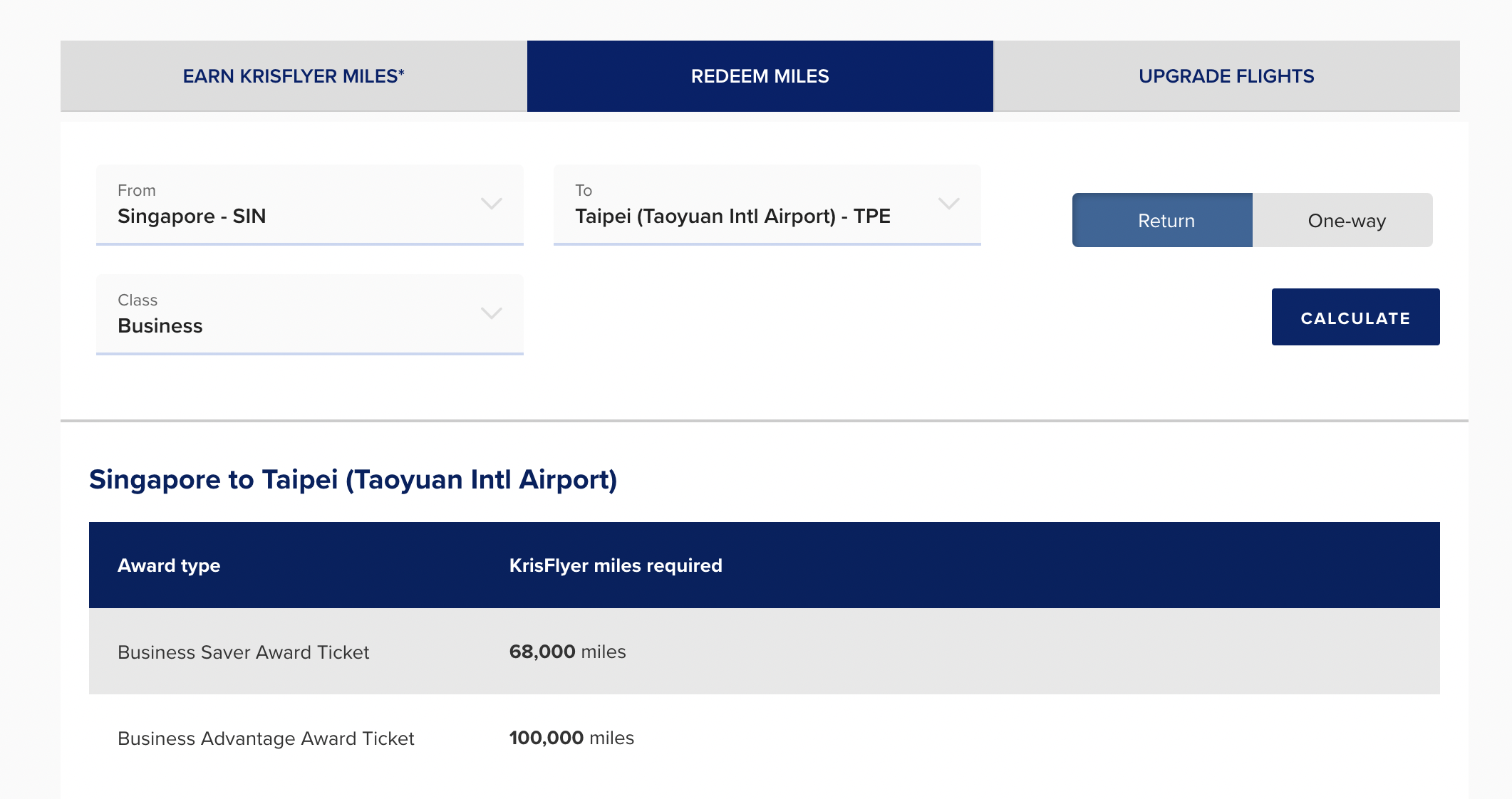The image displays a user interface for booking flights using miles. The layout is structured and color-coded for clarity. 

1. **Header Section:**
   - On the left, a light gray box labeled "Earn Chris Flyer Miles" with blue text.
   - In the center, a dark blue box with white text titled "Redeem Miles."
   - On the right, another light gray box that reads "Upgrade Flights" in blue text.

2. **Flight Search Section:**
   - Below the header, fields for flight route selection appear:
     - "From Singapore (SIN)", with a drop-down arrow for selection.
     - "To Taipei (Taoyuan International Airport) (TPE)", also with a drop-down arrow.
   - Next to the route, there is an option for "Return", which appears to be highlighted.

3. **Calculation Section:**
   - A button labeled "Calculate" is present.

4. **Class and Route Details:**
   - On the left, under the "Calculate" button, it states "Class: Business" with a drop-down arrow for class selection.
   - Directly beneath, it restates "Singapore to Taipei (Taoyuan International Airport)".

5. **Award Type and Miles Required:**
   - This section details the miles required for different types of award tickets:
     - "Award Type: Chris Flyer" shows that it requires different mile amounts.
     - The "Miles Required" part is highlighted in dark blue. 
     - "Business Saver Award Ticket (68,000 Miles)" is shown in a light gray highlight.
     - "Business Advance Award Ticket (100,000 Miles)" is displayed with a white background for clarity.

This structured UI seems designed to help users easily navigate and select their preferences for redeeming flyer miles on the Singapore to Taipei route.